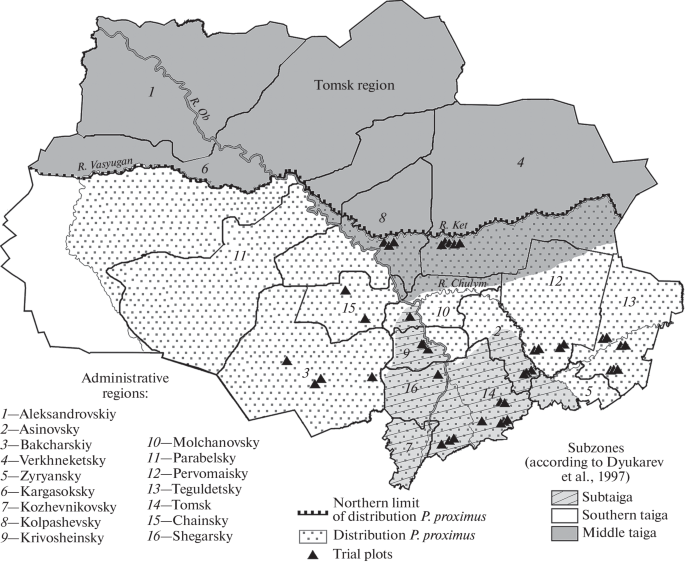The image is a black and white map from 1997 titled "Administrative Regions of the Czech Republic." The map itself dominates the center, stretching from left to right, and is not shaped like any familiar country outline. It is divided into 16 regions, each labeled with a number and name, such as Aleksandrovsky, Asanovsky, and Bakcheresky. In the top left corner, there is a section labeled "Tomsk Region." The map includes various text labels such as "Northern Limit of Distribution," "Distribution," "Trial Plots," and "Subzones according to the Darn Curve," with the different subzones marked as "subtaiga," "middle taiga," and more. These areas are visually represented in shades of white, gray, and black, with dots and lines indicating specific features. A legend at the bottom right corner explains these visual markers, including triangles that denote trial plots.